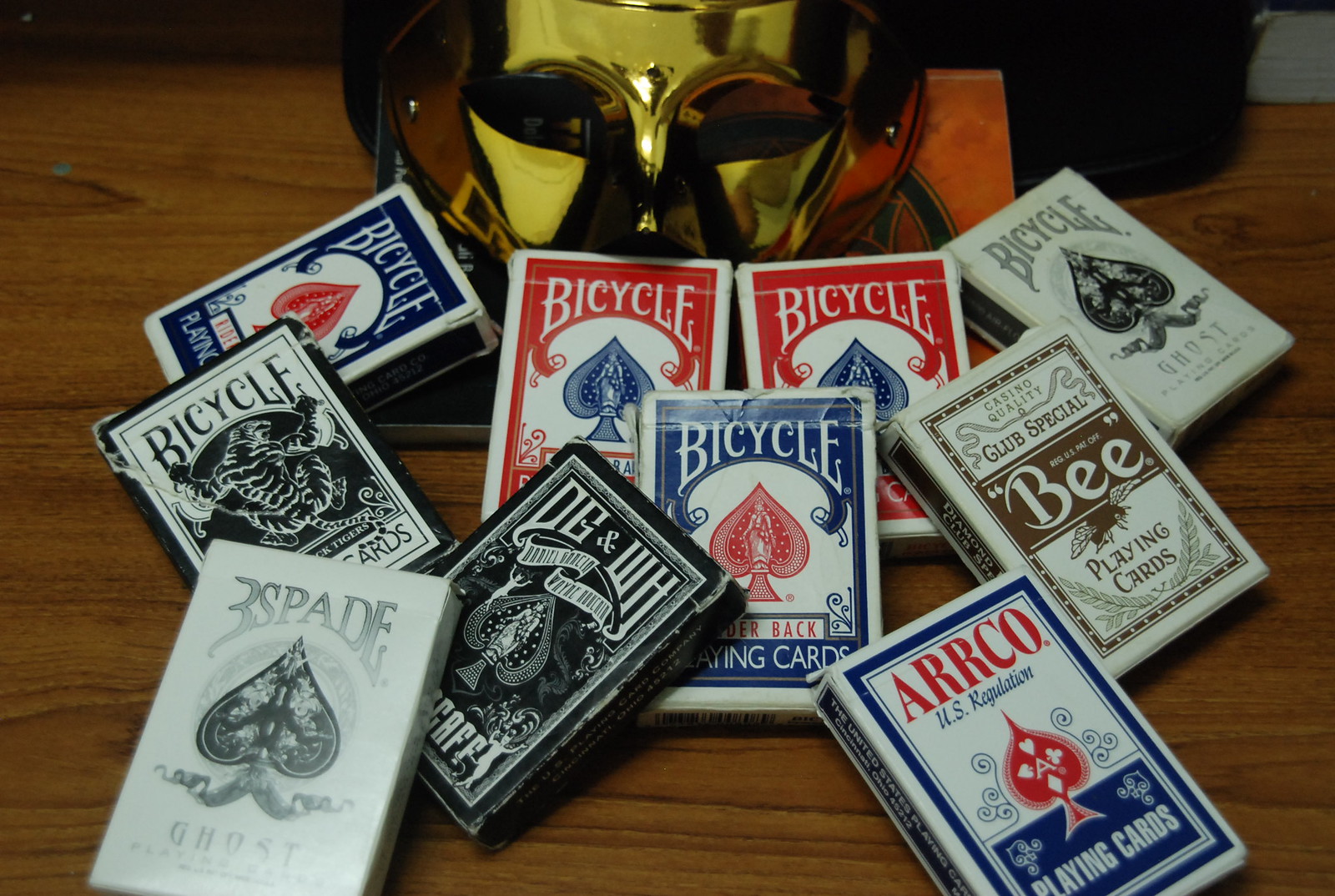This photograph features an intricate arrangement of ten decks of playing cards, meticulously positioned in front of a striking gold mask. Dominating the center of the image are two prominent packs of Bicycle cards, primarily red with a distinctive blue spade design at the top. Flanking these central decks are additional Bicycle cards: to the left, a white pack adorned with a black spade, and to the right, a blue pack with a red spade.

Below these, another Bicycle deck is showcased, this one featuring an intriguing illustration of a creature—possibly a tiger—scratching beneath the Bicycle logo. Adjacent to this, further down, is a white deck with a large, bold spade on the front. Close to the center, but slightly to the right, is a blue pack of cards marked with the letters "D, G, and W, H," also sporting a prominent spade.

The exact center of the display holds another Bicycle pack, this one with a red spade. Positioned on the right side of the tableau is a distinctive black and white deck labeled "Casino Quality Club Special Bee," with a notable "B" visible below the word "Bee." Finally, at the lower right corner, there is an ARCO deck, identified by its red spade and a blue rectangle indicating "playing cards." All these packs rest on a wooden table, angled upward to directly face the viewer, with the gold mask serving as a dramatic and elegant backdrop.